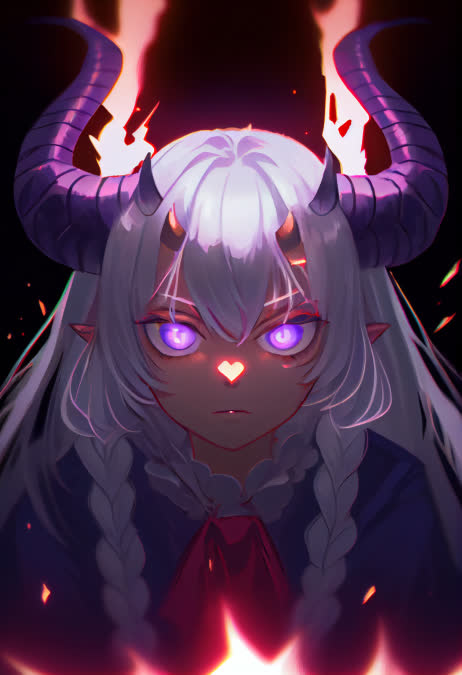In a striking anime-style illustration, a girl with an alluring yet serious expression dominates the scene. Her long white hair is elegantly styled into a couple of braids, and she gazes directly at the viewer with mesmerizing, vibrant purple eyes. The most remarkable feature is her multitude of horns: three pairs in total. The smallest pair, a vivid red, sits just above her eyes, followed by a slightly larger but still small pair positioned higher and wider. The largest, most impressive pair are fully developed, curving majestically upwards and outwards from the sides of her head. Complementing her distinct appearance, she has large, elf-like pointy ears, and a peculiar light heart shape on her nose.

She wears a blue shirt accented by a red scarf draped around her neck, adding a splash of color to her attire. The background is predominantly dark, contrasting sharply with her light figure. Accentuating the drama, it features elements resembling lightning and fire patterns, creating an aura of intensity and power.